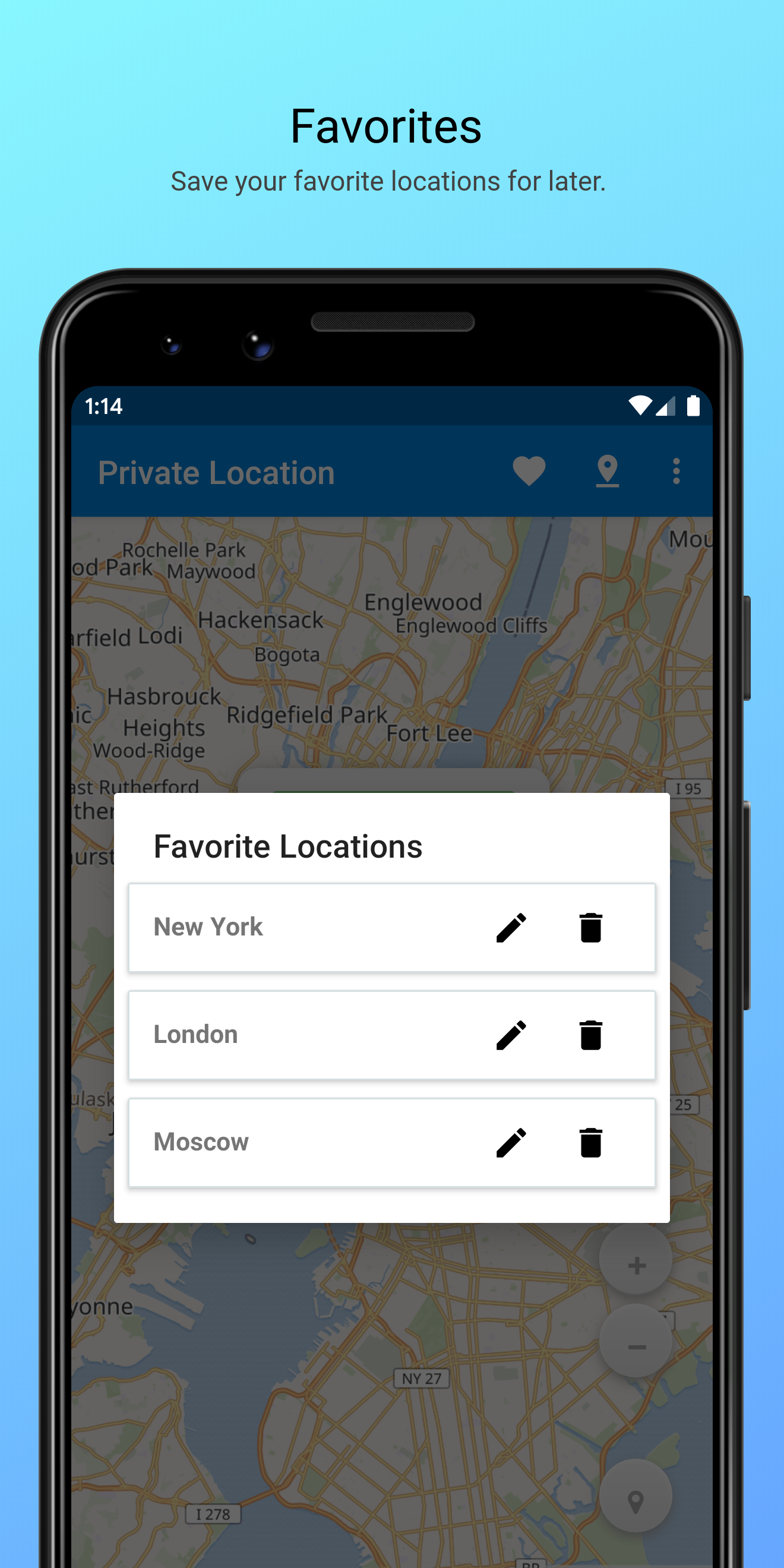The image depicts a smartphone, with its lower portion cut off, against a light blue background. The phone's screen displays a user interface with a "Favorites" section prominently labeled in large, black letters. Below this heading, the text "Save your favorite locations for later." is shown.

The phone itself features a gray border with a black bar at the very top, followed by a blue status bar displaying computer icons, the current time on the left, and other standard icons on the right. Beneath this, the display shows the label "Private Location" in white text, accompanied by a heart icon, a search icon, and a three-dot menu icon to the right.

The main area of the screen is occupied by a map highlighting various streets, towns, and a central water feature, which appears to be a river or bay.

Centrally positioned on the map is a white overlay box, labeled “Favorite Locations” in black text. Inside this box, three location entries are listed: "New York," "London," and "Moscow." Each entry has an edit (pencil) icon and a delete (trash can) icon on the right side for managing the saved locations.